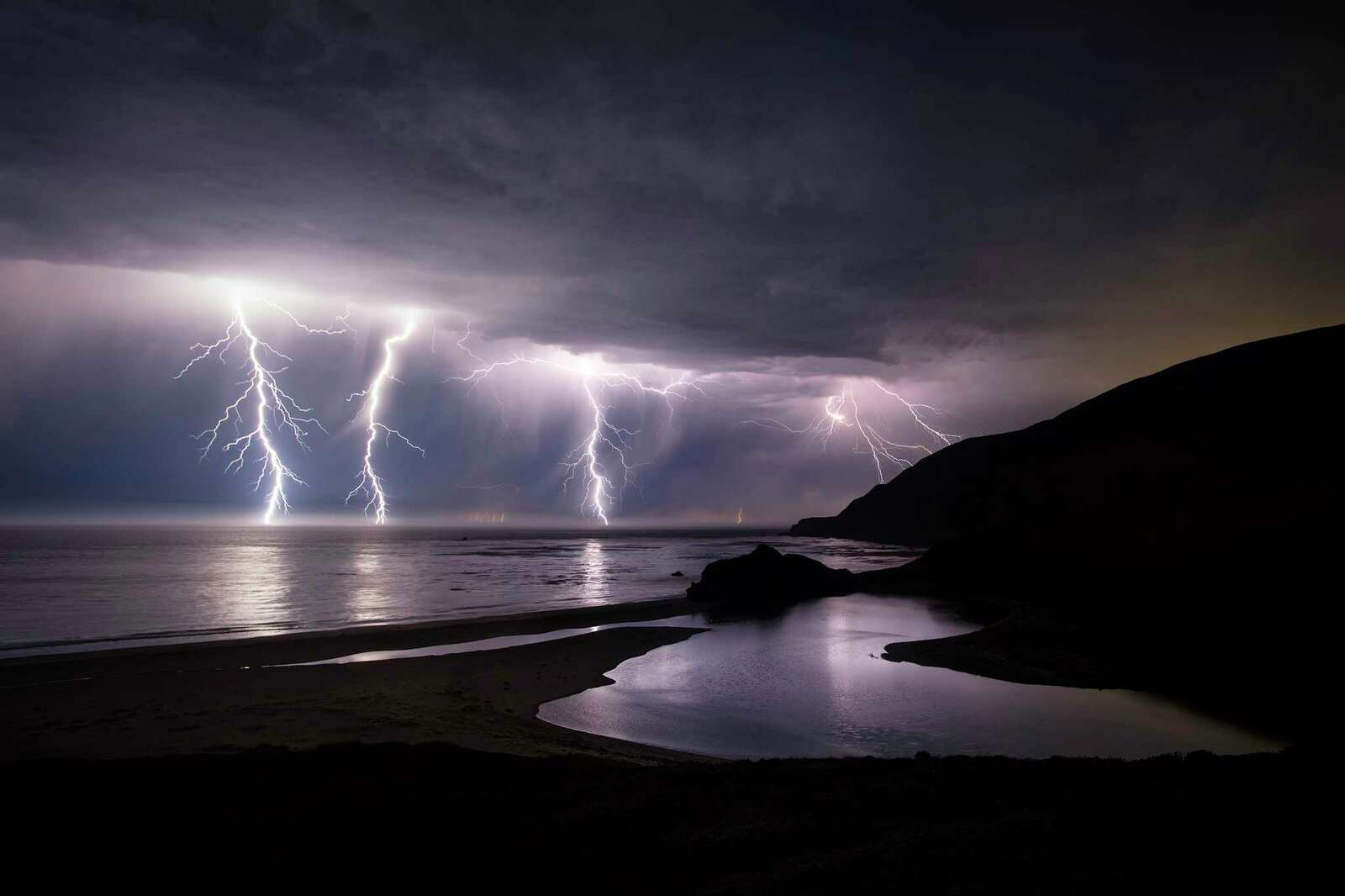This photograph captures a dramatic nighttime thunderstorm over a calm sea, viewed from a beach. The sky is dominated by thick, dark storm clouds, punctuated by four vivid and powerful lightning bolts that illuminate the scene. These lightning bolts create a radiant white and purple glow, making the clouds and falling rain visible against the otherwise dark sky. The waters of the sea are calm and reflective, mirroring the lightning's light. To the right, the silhouette of a hill frames the scene, creating a sense of being in a cove or valley. On the left, the faint trace of a light tan sandy beach is just visible. The overall composition beautifully contrasts the serene, dark waters with the intense, electrifying storm above, highlighting the natural power and beauty of the environment.